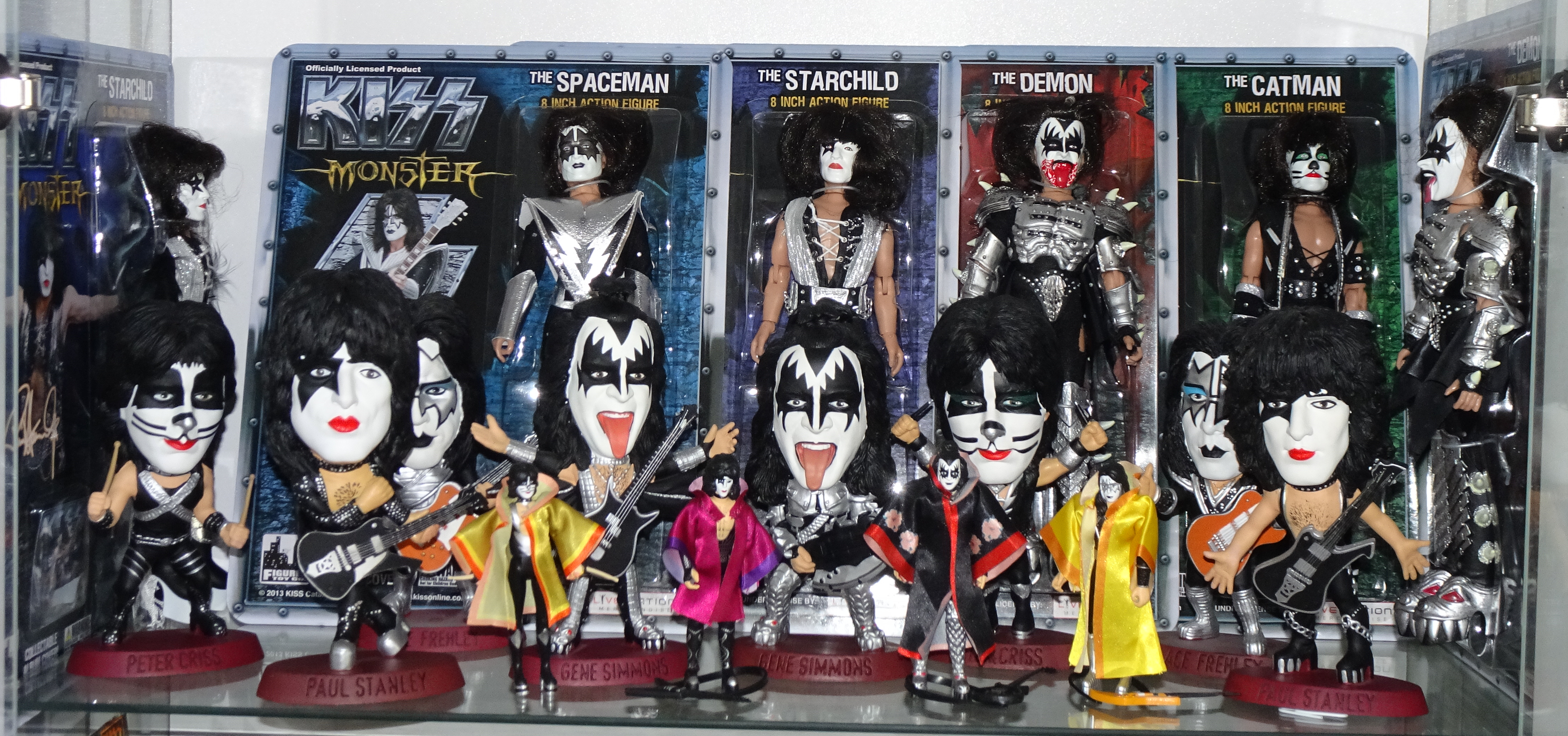The image is a horizontally oriented, slightly angled color photograph showcasing a single glass shelf filled with meticulously arranged KISS memorabilia against a plain white wall. The back of the shelf features several action figures of the band members—The Spaceman, The Starchild, The Demon, and The Catman—still in their original plastic display cases with metallic font labels identifying each character and the word "MONSTER" in yellow. In front of these boxed figures are six to eight KISS bobbleheads displaying the same iconic black and white makeup, each on a base with text indicating the member's name. The front row consists of smaller KISS figurines, each with distinctive black and white face paint and red tongues prominently sticking out, capturing the band's signature look. The entire display appears to be a prized collection, carefully curated to showcase a variety of KISS-themed items.